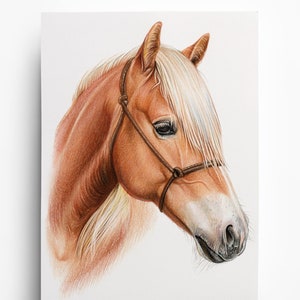This is a detailed photograph of a hand-drawn illustration on a white canvas board, which is attached to a plain white wall, casting a subtle drop shadow on the left, indicating it is slightly hanging off the wall. The painting features an intricate side-view of a horse's head and neck positioned towards the right side of the canvas. The horse, predominantly brown, exhibits a mixture of white and dark gray near its closed mouth, alongside black lips and dark eyes. Golden blonde, somewhat shaggy hair tops its head, partially covering its eyes. Prominent in the artwork are brown straps that run behind the ears and over the nose, likely part of a bridle or muzzle. The horse's tall ears and the meticulous detailing on the headgear further enhance the lifelike quality of this artwork—a refined blend of colored pencils or pastel, executed with exceptional skill but unsigned by the artist.